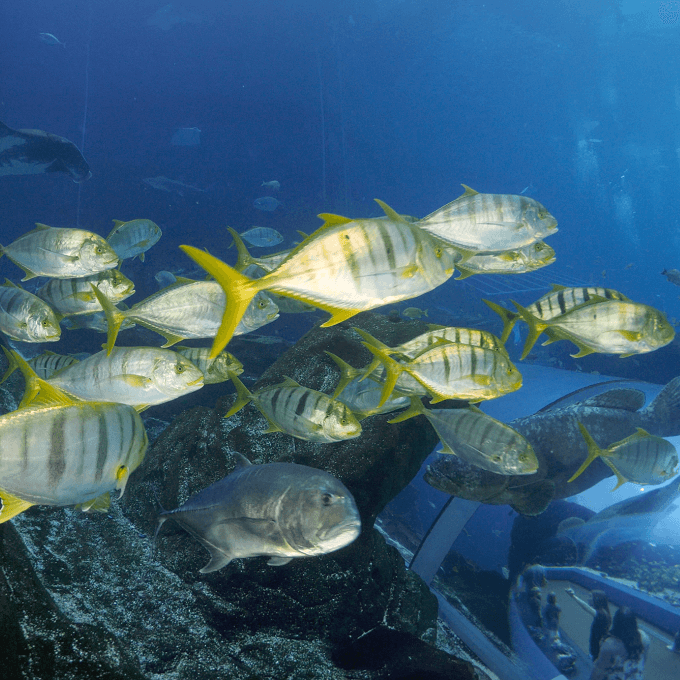This underwater photograph showcases a dynamic scene filled with life and vibrancy. The image, set in a deep blue ocean, captures the mesmerizing play of light and contrasts. Rays of light pierce through the upper right, contrasting with the darker blue tones that dominate the lower left. Here, a large, lightly blue-toned rock rests, adorned with moss and providing a habitat for marine life. Swimming in the foreground is a school of strikingly striped fish, primarily silver with vertical green stripes, bright green eyes, and green fins. They also have notable black stripes down their bodies and vibrant gold tails and gills, adding to their vivid appearance.

Highlighted in the lower right corner is an underwater observatory or submarine, featuring a large glass pane through which families, including both children and adults, are visible, absorbed in observing the underwater spectacle. The tube structure, possibly plexiglass-covered, offers a unique vantage into this aquatic world. Additional marine life, including a larger grey fish speckled with white spots, reminiscent of a coelacanth, and even a hammerhead shark, can be seen in the background, bridging the elements of an aquarium-like setup with the authentic expanse of the ocean. The scene brilliantly captures the interplay between natural marine habitats and human curiosity, framed in a square photograph that invites endless fascination.